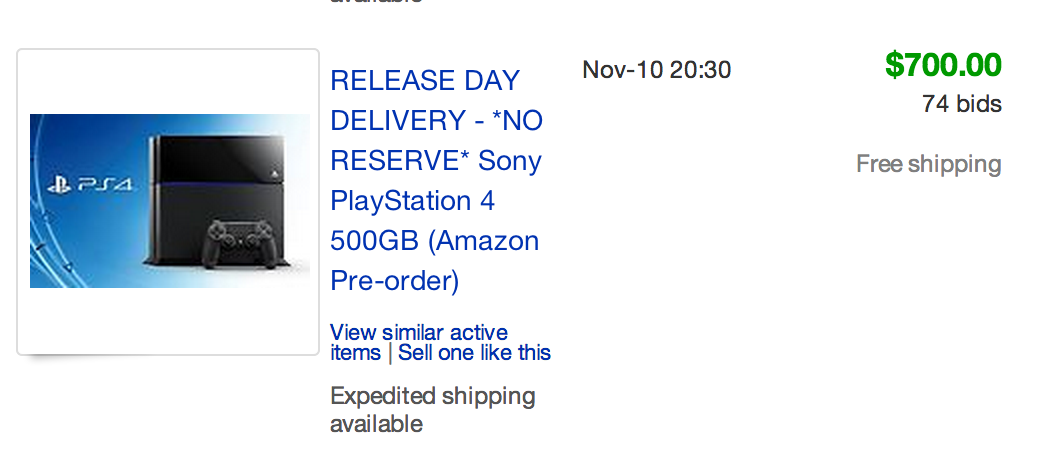Caption: 

This image is a detailed screenshot from an online auction site, likely something like eBay. It features a brand new Sony PlayStation 4 with a 500GB capacity, prominently displayed on the left side of the screen. The PlayStation 4 listing is particularly notable for its "Release Day Delivery" and comes with no reserve, signifying a potential bargain for bidders. The product was listed as an "Amazon Pre-Order," highlighting its anticipated demand. An array of textual elements reads, "Release Day Delivery, No Reserve, Sony PlayStation 4, 500GB, Amazon Pre-Order, View Similar Active Items, or Sell One Like This, Expedited Shipping Available, November 10, 2030." The auction has garnered substantial interest with 74 bids pushing the current price to $700, and free shipping is included to sweeten the deal. The webpage itself has a simple, clean white background, emphasizing a professional yet user-friendly auction platform designed for both sellers and buyers.